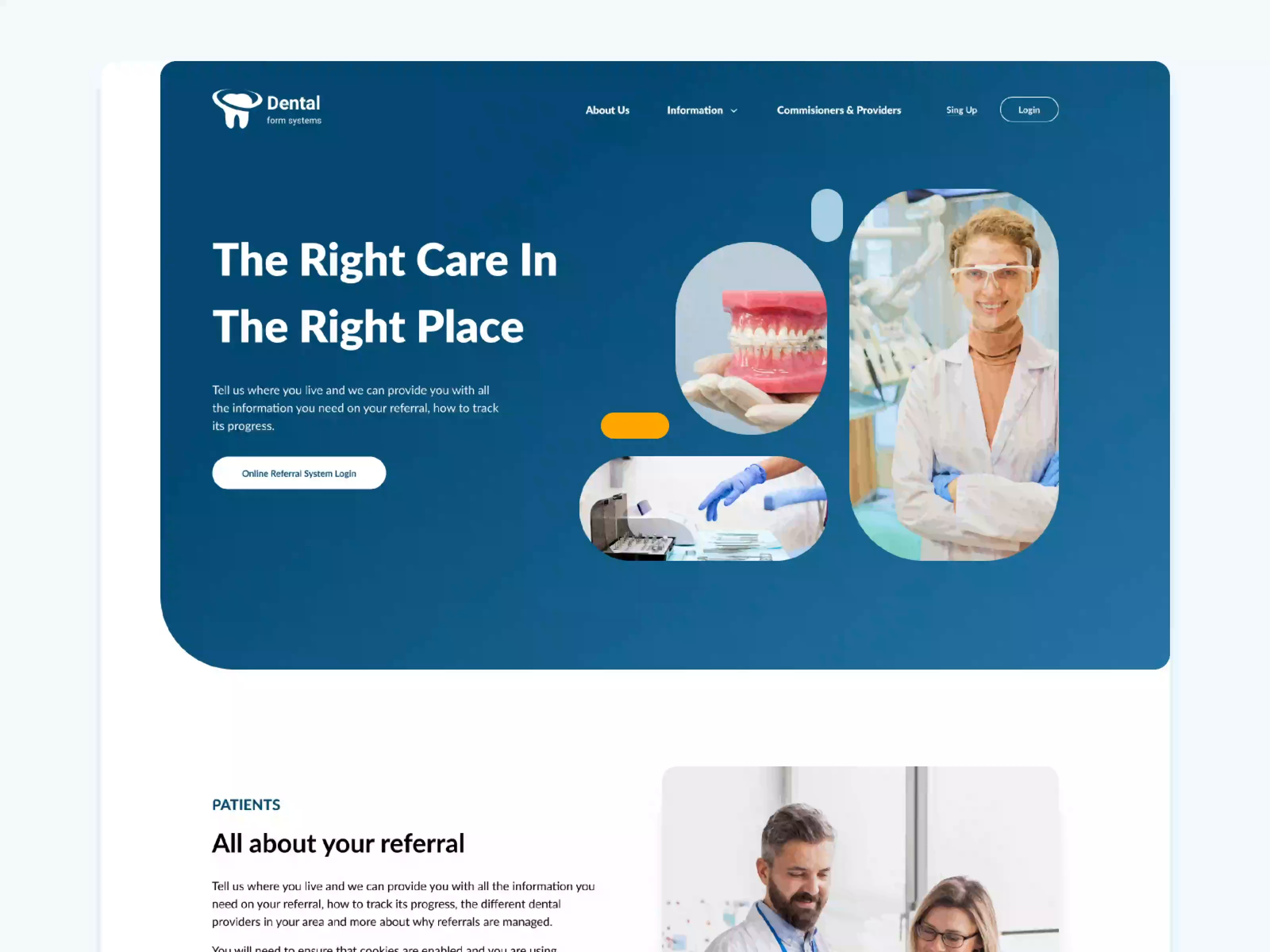**Detailed Caption:**

The image features a comprehensive online dental referral system presented on a clean interface with a blue background and white text. At the top, the tagline "The right care in the right place" is prominently displayed. The website instructs users to "Tell us where you live," promising to provide all necessary information about their referral and track its progress.

In the center of the image is an online referral system login page surrounded by three distinct visual elements. On the left, there is an oval-shaped photo where a person, wearing white gloves, is holding a tooth model. The model displays pink gums and white teeth, reminiscent of a tooth-chattering toy, emphasizing the dental aspect of the service.

In the middle image, just below the first, another person, this time with blue gloves, is seen hovering their hands over some intricate dental instrument or device, showcasing the precise and detailed nature of the equipment used in dental care.

To the right, a third image features a professional woman dressed in a white lab coat and a turtleneck, sporting safety glasses and blue latex gloves. She stands confidently with folded arms, and behind her, a piece of dental machinery can be seen, highlighting the advanced technology used in the service.

Above these images, an "About Us" section with a drop-down box for additional information, alongside buttons for Commissions, Sign Up, and Login, is visible. Below the images, a section labeled "Patients" in blue, with "All about referral" written beneath, provides additional details to users about the referral process. Another call to action repeats, "Tell us where you live. We can provide you with all the information you need on your referral."

Towards the bottom of the image, a partial depiction shows a doctor or dentist consulting with a patient who is wearing glasses, though the image is slightly cropped, emphasizing the personalized care approach of the service.